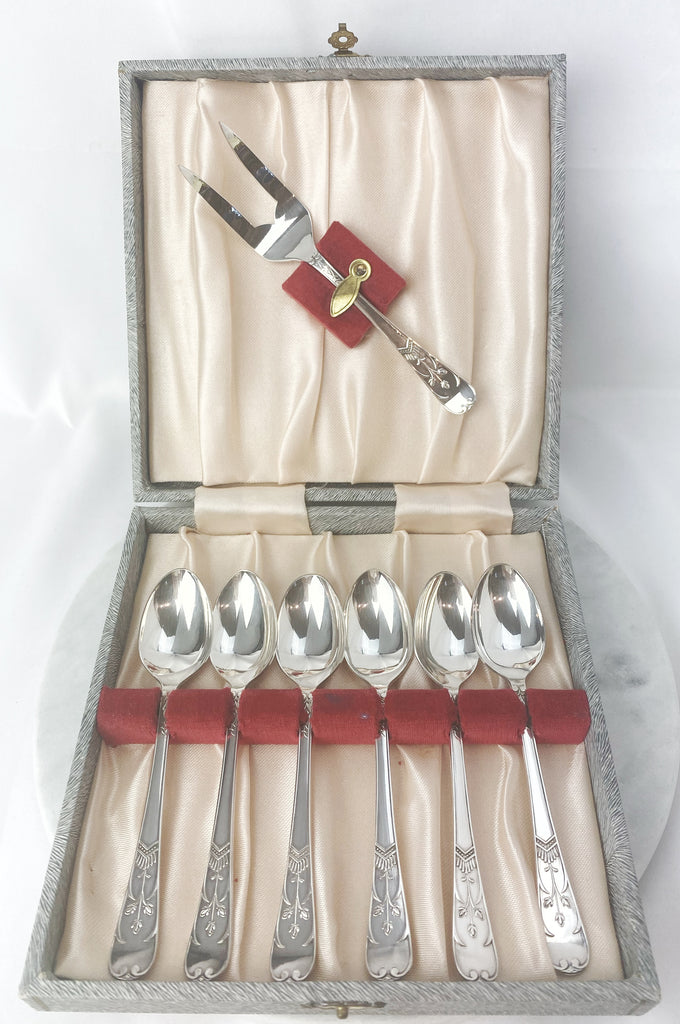The image depicts a gray box set against a marble-like background, designed to hold and protect sterling silver dining ware. Inside this elegant case, the base section showcases six meticulously arranged silver spoons, each nestled in individual red velvet slots. The spoons are small, with shiny, slender necks that widen into intricately decorated bases featuring floral designs. A layer of cushioned satin tan fabric lines the box, adding an extra touch of sophistication and protection. The upper part of the box reveals a shiny silver serving fork with two prominent prongs, secured by a gold clasp against a matching red velvet background. This luxurious presentation is complemented by the satin lining on the lid, harmonizing with the overall opulent appearance of the set.